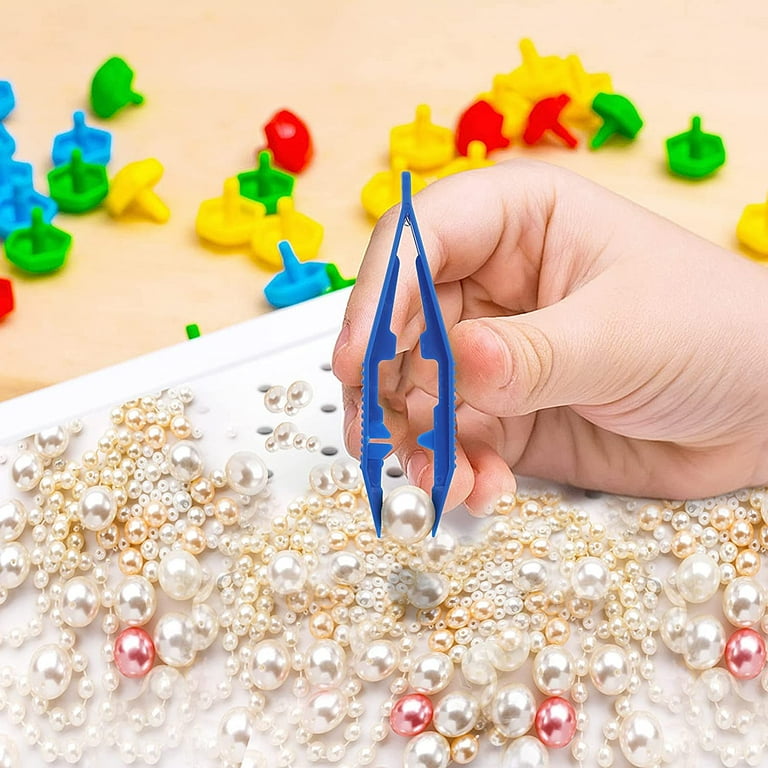The image depicts a right hand, fair-skinned, holding a pair of blue tweezers and picking up a white pearl-like bead from a tabletop scattered with various beads. These beads are of different sizes and colors, primarily white with some pink, smaller gold-tinted ones, and a few red ones. The tabletop itself is white with perforated holes in a pattern. In the background, various colorful plastic game pieces resembling simple spinning tops in blue, green, yellow, and red are visible, adding to the scene's playful atmosphere.